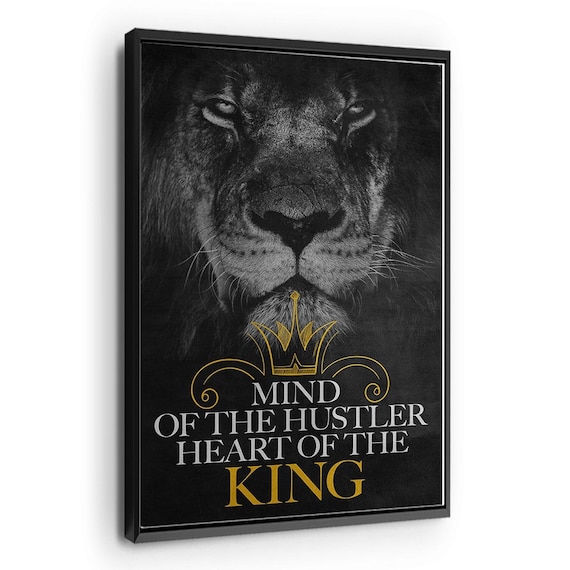The photograph captures an intricately designed motivational poster encased in a black picture frame, slightly tilted to the left against a white wall backdrop. At its center is a realistic, black-and-white close-up of a lion's face, exuding a fierce and determined expression, its eyes, nose, and mouth vividly detailed while its surrounding fur gradually fades into darkness. Below this powerful image, set against the black background, is the inspirational text, "Mind of the Hustler, Heart of the King." The text is primarily written in white, except for the word "King," which stands out in a striking gold font. Positioned above the text is an elegantly drawn, golden crown adorned with a central spike that features a gold diamond shape on top. The crown displays French-inspired decorative curls at its base, adding a sophisticated touch to the bold message. This beautifully crafted motivational piece, designed to inspire determination and strength, is framed with a black border accentuated by a white outline, making it a striking item for any space intended to evoke empowerment.